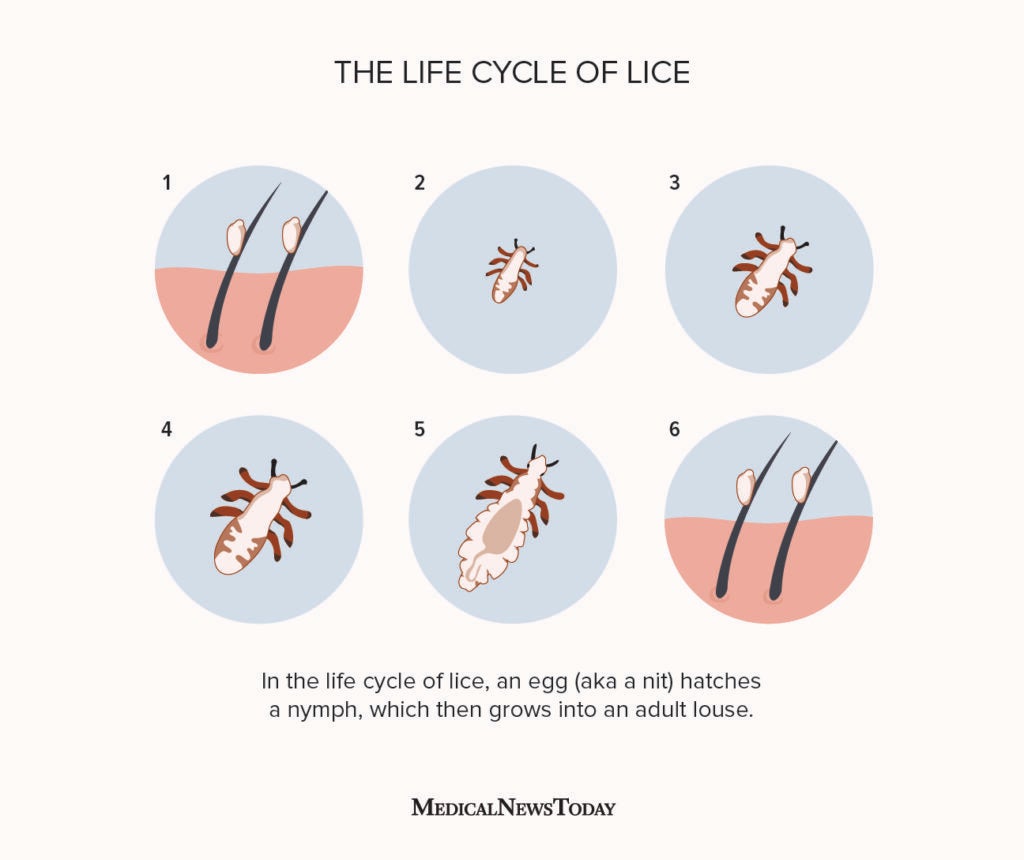The illustration titled "The Life Cycle of Lice" presents an informative infographic detailing the six stages of lice development. The sequence is depicted in six circles, each with a light blue background and numbered 1 to 6 in the top left corner. 

In the first and sixth circles, the bottom half is pink, representing skin, with two hair follicles emerging, each hosting a tiny white egg, or larva. The second circle shows an isolated nymph, slightly larger than the eggs, with a white body, six brown legs, and two dark antennae pointing diagonally upward to the right. 

The third and fourth circles depict the nymph growing progressively larger, retaining the six legs, two antennae, and developing small brown triangular markings along its abdomen. By the fifth circle, the lice is shown as an adult, noticeably larger, with a distinct light tan lozenge on its back and a fatter, segmented abdomen, indicating full maturity.

Beneath these images, text explains: "In the life cycle of lice, an egg (also known as a nymph) hatches a nymph, which then grows into an adult louse." At the very bottom, the source "Medical News Today" is credited in bold, capitalized text. Overall, the design conveys the continuous growth cycle of lice, from egg to mature adult, emphasizing the persistent nature of these parasites.